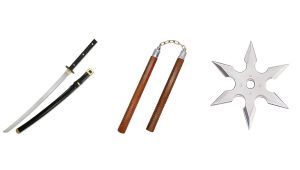The image presents three different Asian weapons on a plain white background with no text. On the left, there is a katana, characterized by its black handle with white dots and its silver blade, lying next to a black sheath adorned with gold trim. In the center, there is a pair of wooden nunchucks, connected by a metal chain, featuring silver metal tips. To the right, there is a highly polished, six-pointed, silver ninja star with a circular cutout in the middle, clearly sharp and designed for throwing. The weapons are likely not to scale, especially as the ninja star appears almost as large as the katana.